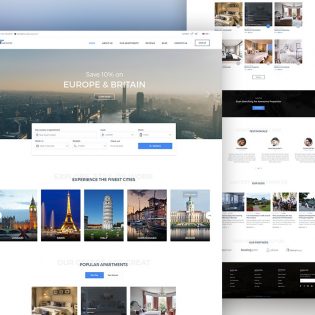A travel website is displayed, comprising two overlapping pages viewed from a distance, making the text difficult to read. Prominent promotional text offers a 10% discount on trips to Europe and Britain. The webpage features iconic images, including the Eiffel Tower and the Leaning Tower of Pisa, alongside other less recognizable landmarks. One page appears dedicated to customer reviews of the travel services, while another section highlights popular accommodations, suggesting it may assist users in finding places to stay or planning their trip to Europe and Britain.